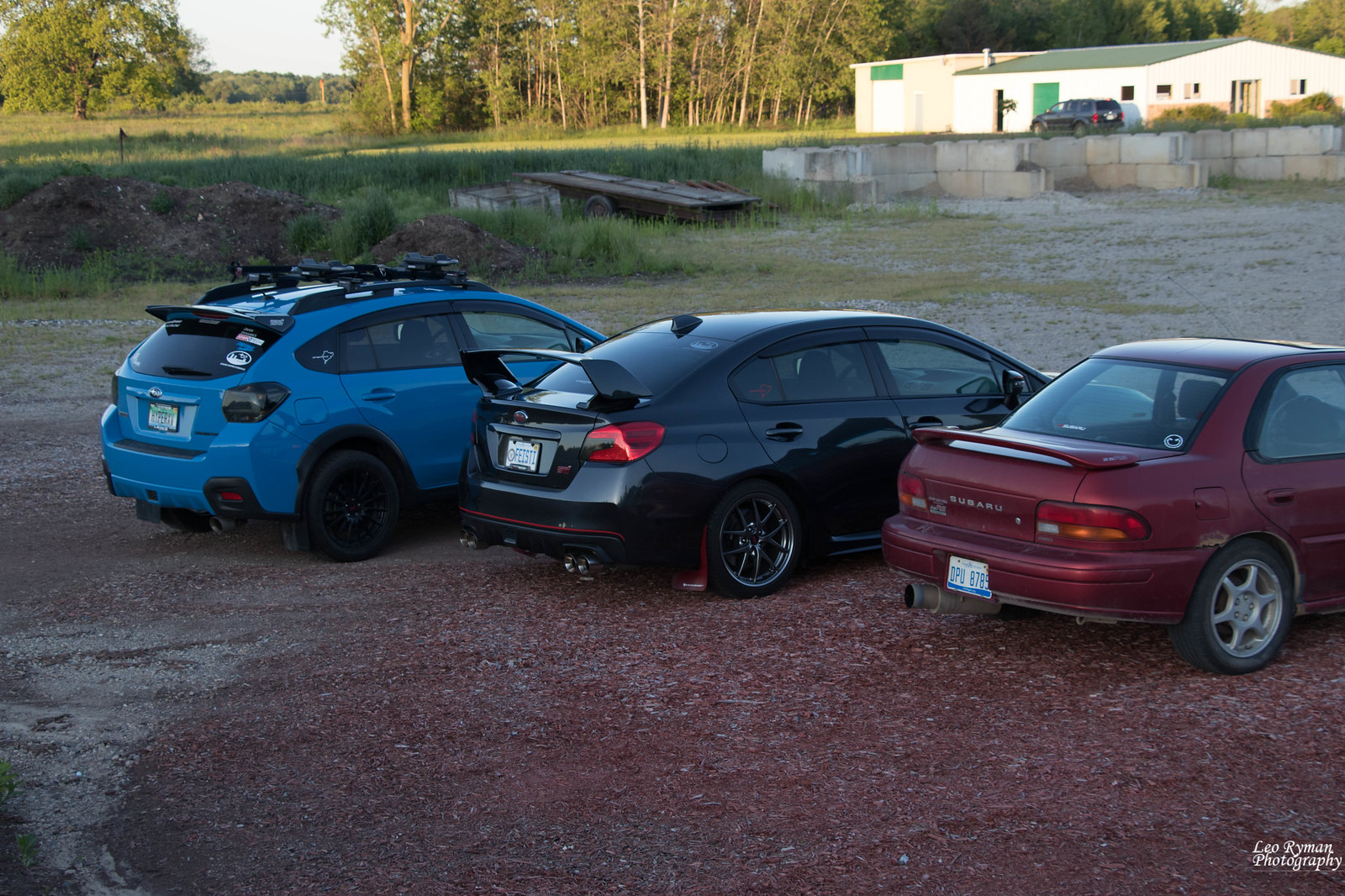The photo depicts an outdoor scene featuring three different cars parked side by side on a gravel parking lot. To the left, there's a blue five-door car, somewhat resembling a chopped-up sedan, equipped with a roof rack. In the center, a sleek black Toyota sedan sports a spoiler and black rims. On the right, a vintage red Subaru sedan from the mid to late 90s completes the trio. The backdrop includes a sprawling sky with light blue hues and a densely wooded area with bright green foliage on the left and various tree types with brown and white trunks stretching to the center. A white building with a green door and a cylindrical concrete structure topped with a van are visible to the right. The image bears a small watermark in the bottom right corner that reads "Leo Ryman Photography," emphasizing its professional origin.